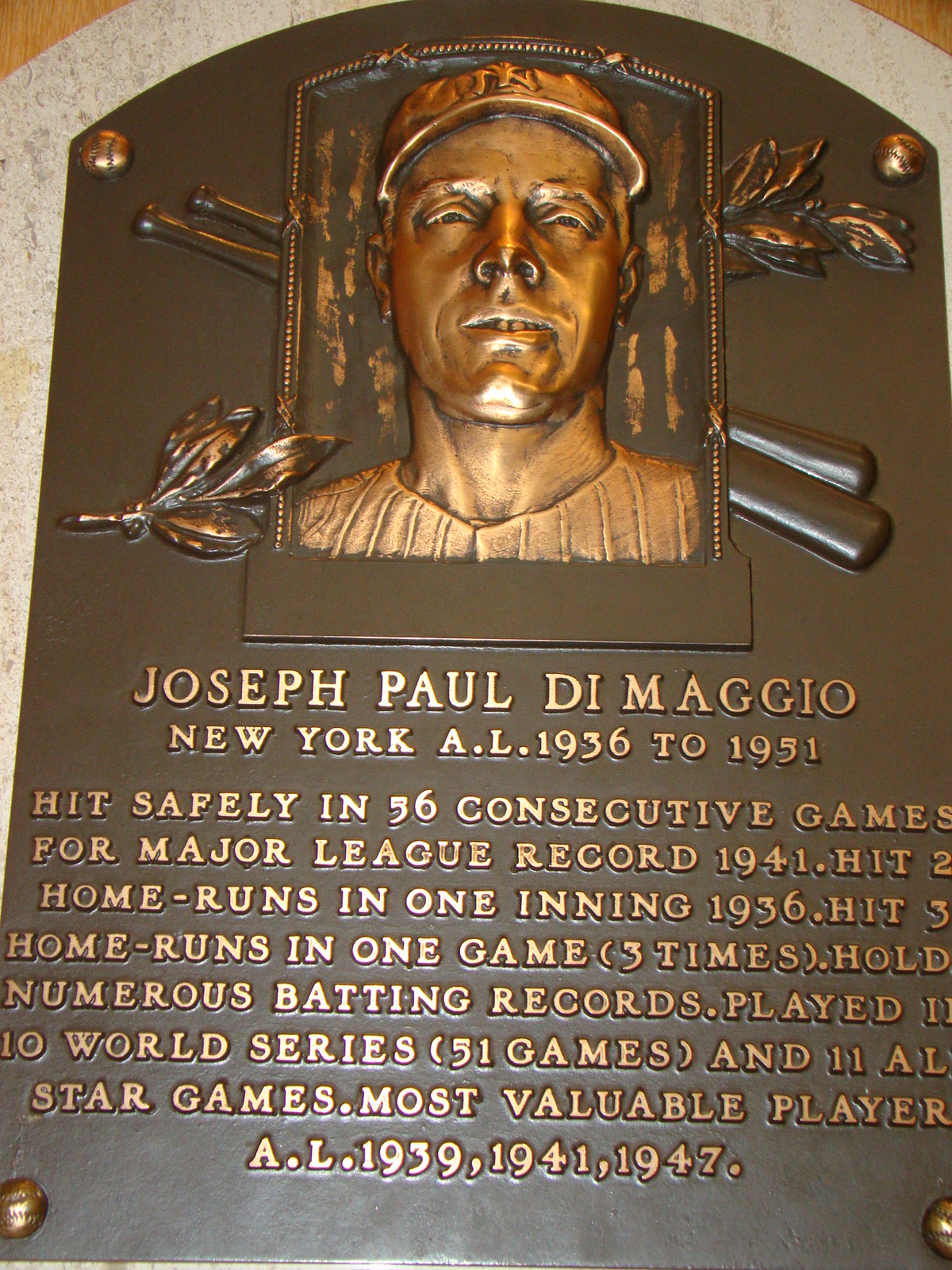This image prominently features a detailed bronze plaque honoring the legendary baseball player Joseph Paul DiMaggio. The plaque, likely displayed at either the Baseball Hall of Fame or Yankee Stadium, fully occupies the frame, leaving no background visible. At the top, a bronze relief of DiMaggio's face is depicted, wearing a Yankees cap. Surrounding the image are two crossed baseball bats and delicate gold leaves, adding to the plaque's ornate design. The text, in raised yellow letters, chronicles DiMaggio’s illustrious career: "Joseph Paul DiMaggio, New York, AL, 1936-1951." Key highlights include his record-setting 56 consecutive games with a hit in 1941, hitting two home runs in a single inning in 1936, achieving three home runs in one game on three occasions, and holding numerous batting records. DiMaggio's impressive participation in 10 World Series (51 games) and 11 All-Star games, along with his titles as the American League's Most Valuable Player in 1939, 1941, and 1947, are also noted. The plaque features colors of bronze, black, brown, and white, giving it a rich, historical feel. Small gold circular buttons adorn the upper right and lower left corners, adding to its distinguished appearance.